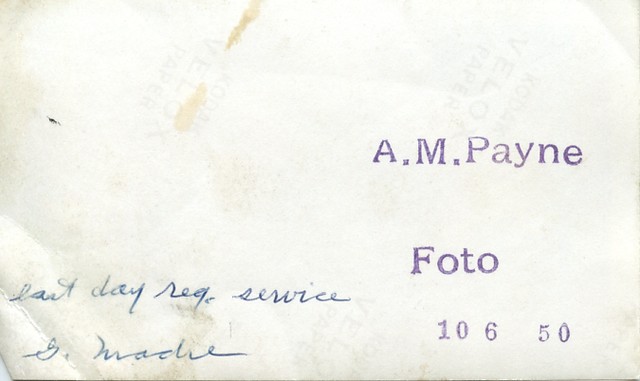This photograph captures a weathered piece of paper with notable characteristics. At the top, there are prominent brown stains accompanied by a stray black mark. On one side of the image, a handwritten note reads "Last day of regular service," followed by what appears to be someone's signature. Opposite to this note, in a dark-colored font, the text "A.M. Pain FOTO 10 650" is visible. The paper shows the faint outline of dark-colored text that is printed on the reverse side, suggesting some transparency. Additional brown stains are scattered towards the bottom of the paper, and the corners are visibly wrinkled. Subtle shadowing around the edges emphasizes the aged and fragile nature of the paper.